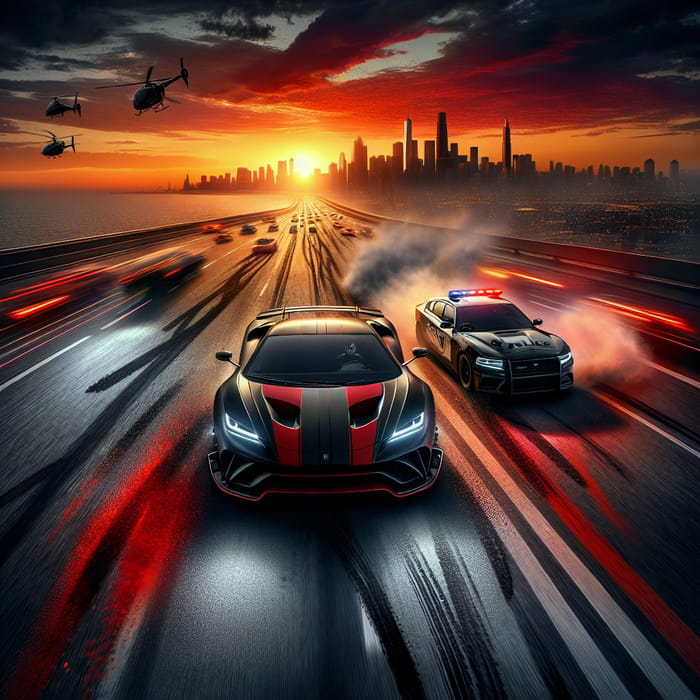This square-shaped artwork, measuring approximately five to six inches on each side, vividly depicts a high-speed police car chase on a five-lane freeway emerging from a cityscape at sunset. The upper portion of the image portrays a dramatic sky, with dark gray clouds tinged with orange on their undersides due to the setting sun. The sun itself is a bright white orb encircled by yellow and orange hues. A sprawling city skyline with glowing skyscrapers dominates the horizon, leaning slightly left but mostly extending to the right. Below the sun, a grand bridge stretches out, with water visible to its left and a dark, dotted expanse presumably water or terrain to the right.

In the upper left corner, three helicopters hover against the reddish sky. The central action unfolds on the freeway below, where a sleek black race car marked by two red pinstripes on its hood speeds toward the viewer, leaving trails on the road. Flanking it to the right is a black-and-white police car, its tires smoking and lights flashing blue, a stark contrast to the grayscale and warm tones of the scene. Further back on the freeway are additional cars, adding depth to the chaotic chase. The entire composition, rendered in shades of gray, orange, red, and occasional blues, captures the tension and dynamism of the pursuit.